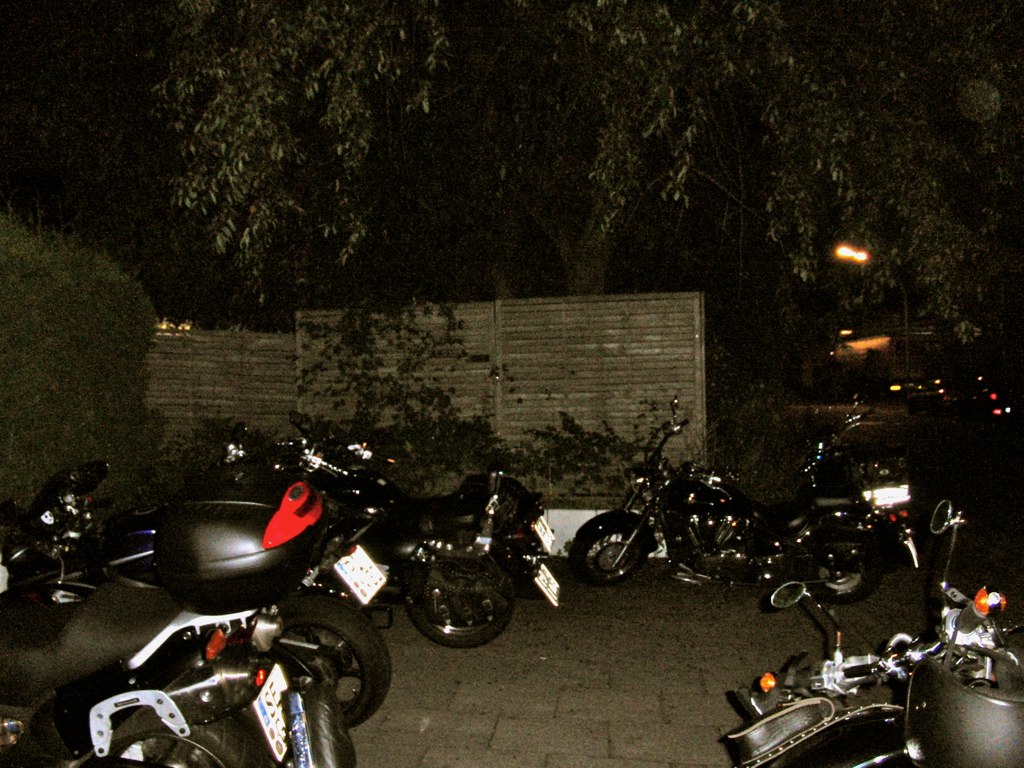This nighttime photograph, taken with a flash, captures a group of motorcycles parked on a large brick-patterned pavement. The foreground showcases an array of motorcycles, predominantly black, with an emphasis on their trunks and high-handlebars adorned with rearview mirrors. One motorcycle features a hint of red at the back. The bikes are parked in a somewhat haphazard arrangement. In the background, a climb of ivy adorns a wooden fence, and beyond that, silhouettes of trees are visible against the faint glow of distant lights from a building. To the left, dense shrubbery and an overhanging tree foliage add texture to the scene. The overall atmosphere suggests a quiet courtyard, possibly a beer garden, with a mix of natural and urban elements.